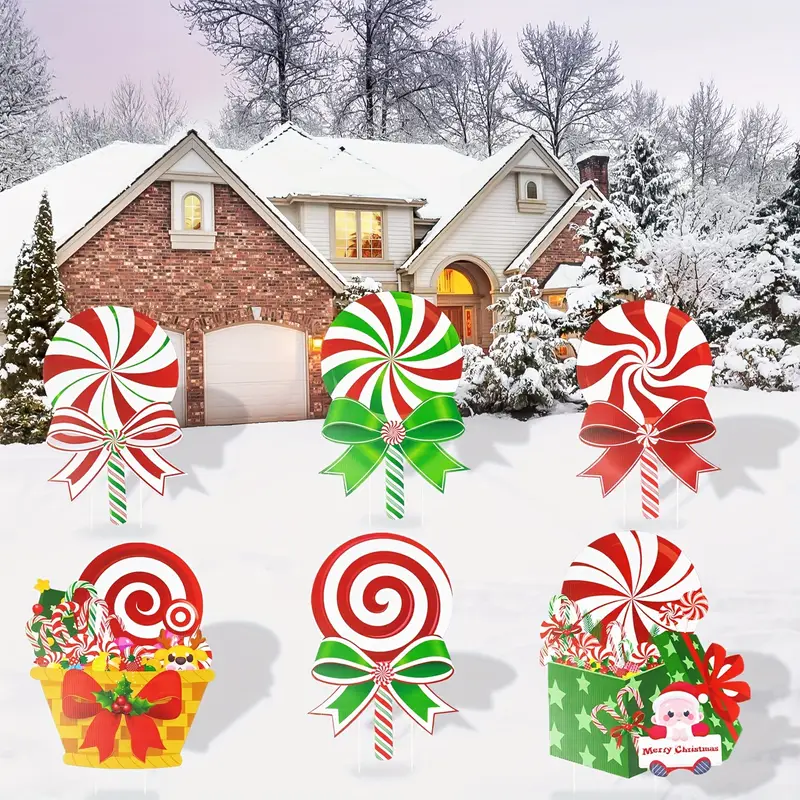This image captures a picturesque winter scene featuring a large, two-story, middle-class family home centered in a snow-covered yard. The house, constructed with red brick and beige vinyl siding, has numerous architectural details including a steeply pitched roof coated in snow, a two-car attached garage with white doors, and a fireplace on the top right. The entire scene is illuminated with a warm, golden light from within the house, suggesting a cozy atmosphere inside.

Surrounding the house are tall trees, both behind and around it, including evergreens that are also blanketed in snow. The driveway, obscured by the thick layer of snow, adds to the sense of a peaceful, untouched winter day.

Overlaying this wintry scene are festive, Photoshopped holiday elements prominently featuring red, white, and green colors: there are illustrated candy canes, mint candies, and popsicles scattered across the bottom of the image. A basket filled with Christmas goodies and a small green gift box complete with a red ribbon and an emblem of Santa Claus holding a "Merry Christmas" sign decorate the bottom right of the image. These cheerful holiday decorations, along with the serene snowy backdrop, give the image the appearance of a holiday postcard or greeting card celebrating the festive season.